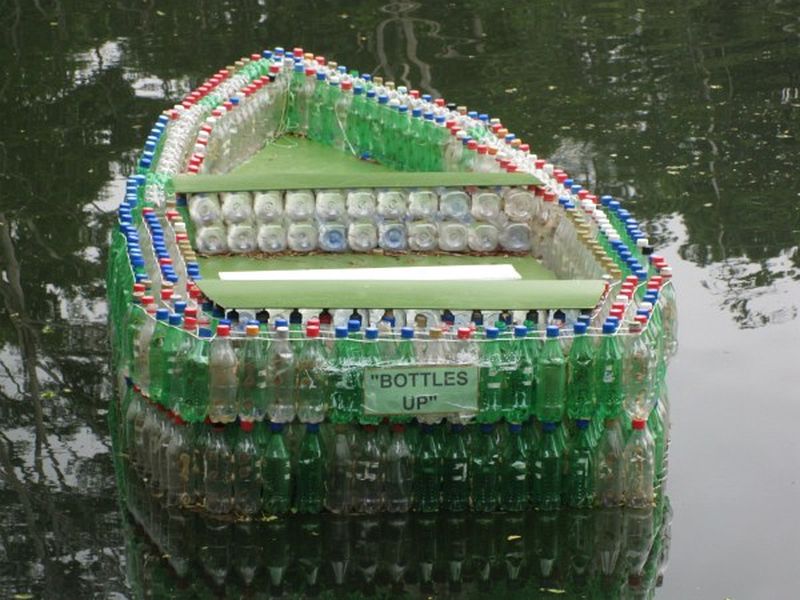The image captures an innovative rowboat ingeniously crafted from recycled 2-liter soda bottles, primarily green ones, likely Sprite, and clear ones that might be Coke bottles. The boat is comprised of rows of tightly secured plastic bottles, arranged in three layers around its edges. The majority of bottle caps are red, white, and blue, with a few yellow and black ones interspersed. The boat is floating on a still, greenish body of water, giving off a serene vibe. A white sign with black text that reads "Bottles Up" is prominently displayed on the back of the vessel. The photograph is taken from an elevated angle, showing the boat from above, with the smooth surface of the water reflecting nearby trees that are not directly visible in the image. Inside the boat, larger bottles form a bench, indicating that one can sit comfortably within this eco-friendly creation.